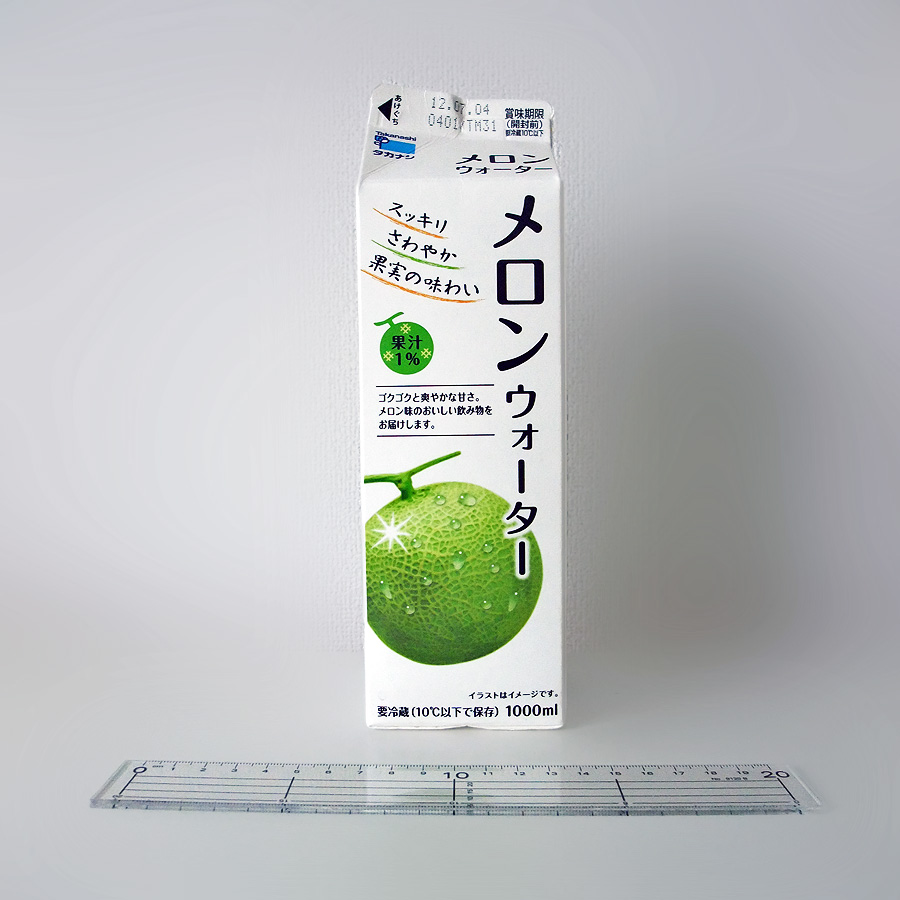This photograph features a tall, rectangular white carton prominently centered against a white backdrop and surface. The carton, adorned with Asian characters—specifically Japanese writing—suggests it contains a type of juice, potentially lime-flavored. The front of the carton showcases a green, rounded fruit resembling a lime, decorated with water droplets and a white star, lending a fresh, dewy appearance. Additional details include black text and colorful accents in green, yellow, and brown. At the top of the carton, an expiry date of 12.07.04 is visible along with the code "0401/TM31". Near the bottom right, it indicates a volume of 1,000 milliliters in black text. Positioned horizontally in front of the carton is a transparent ruler marked in black, measuring from 0 to 20 centimeters, suggesting a setup possibly for an advertisement or product measurement.